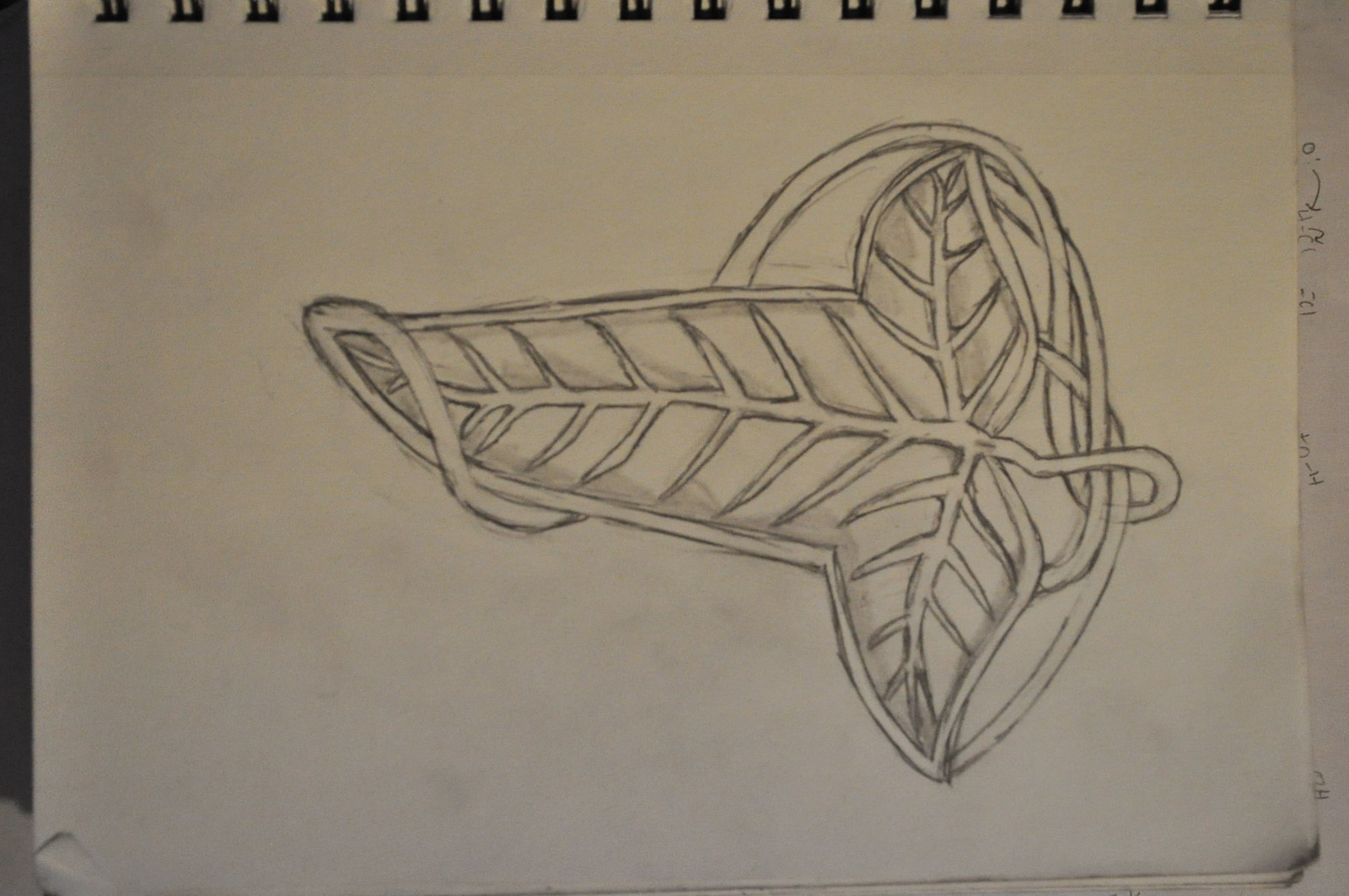The image features an intricately detailed sketch of a large, central leaf with a vine elegantly wrapped around it. The leaf, which has a distinct spine running its length and two smaller side leaves extending from it, is drawn in black and white, likely with pencil or charcoal. The entire sketch is presented horizontally on a slightly off-white sketchbook with a black spiral binding. The longest leaf, positioned toward the left, takes up half the width of the image, while the two smaller leaves extend vertically. The vine winds around the base and the tip of the leaf, adding a dynamic flow to the composition. The drawing occupies most of the page, with smudges at the bottom right edges indicating blending techniques. In the background, to the right of the main sketch, another sheet with math equations peeks out, and the bottom left corner of the sketchbook is slightly bent.